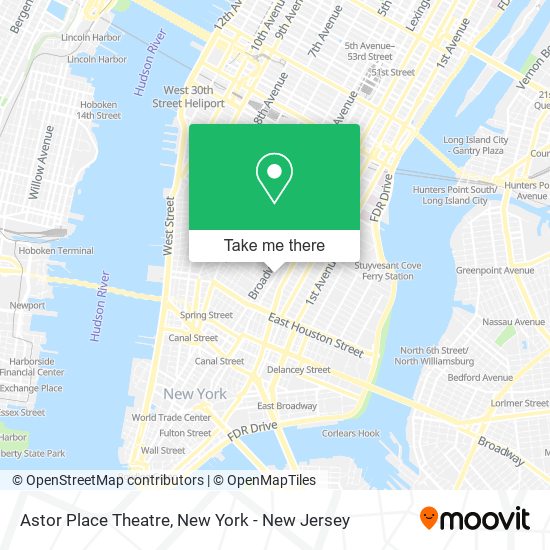This detailed caption describes a screenshot from the Moovit web app, which serves as a navigation tool similar to Google Maps, guiding users through various modes of transportation such as car, train, and walking. The screenshot features a map of Manhattan, New York, with an inset photograph showcasing a building that could be a hotel or department store, located on Broadway just north of East Houston Street. Cars are seen parked in front of the building, with lights illuminating the scene. An arrow points towards the location, and a "Take Me There" button is prominently displayed at the bottom of the inset. Below the map, credits are given to Open Street Map Contributors and Open Map Tiles. The city overlay on the map displays major roads in yellow and detailed street maps in white, with blue shading representing the Hudson River and surrounding waterways. Additionally, the Astor Place Theater is noted as a point of interest in the New York-New Jersey area.